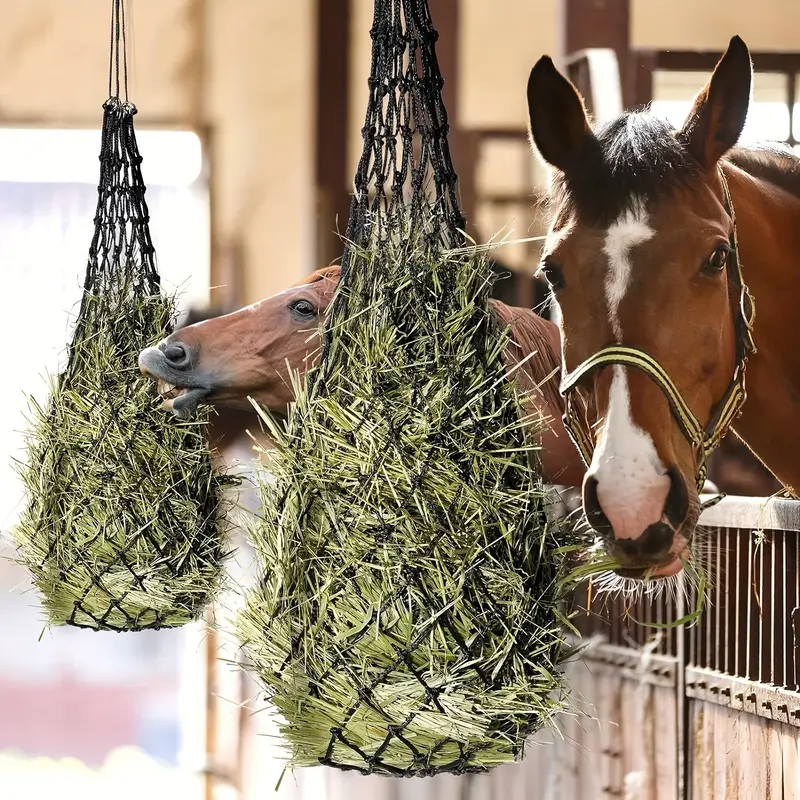This square photograph captures a detailed and vivid scene of two brown horses in their stable, set against a backdrop of cream-colored walls and wooden panels topped with black iron railings. The horse in the foreground, characterized by a white blaze on its forehead and a harness with yellow and black reins, gazes directly at the camera with alert, deep brown eyes, ears perked high. A tuft of hay is visible between its lips, suggesting it has just taken a bite. In contrast, the second horse, positioned slightly behind and to the left, has its head turned away, fully engaged in chewing on hay, and partially obstructed by a net.

Both horses are eating from black, teardrop-shaped nets suspended in front of them. These nets are filled with a mix of green and yellowish hay, with tufts protruding through the netting, which adds texture to the scene. Each horse pulls the hay through the net with ease, illustrating a tranquil moment of feeding.

The foreground horse's reins encircle its neck and nose, adding distinct detail to its appearance. The stable's structure is clearly visible: the wooden panels with rivets constitute the lower part of the fence, while short metal railings with a flat top complete the enclosure. The brightly lit barn interior is warmly illuminated by natural light streaming through a distant door opening to the left and a window on the right, highlighting the peaceful rural setting.